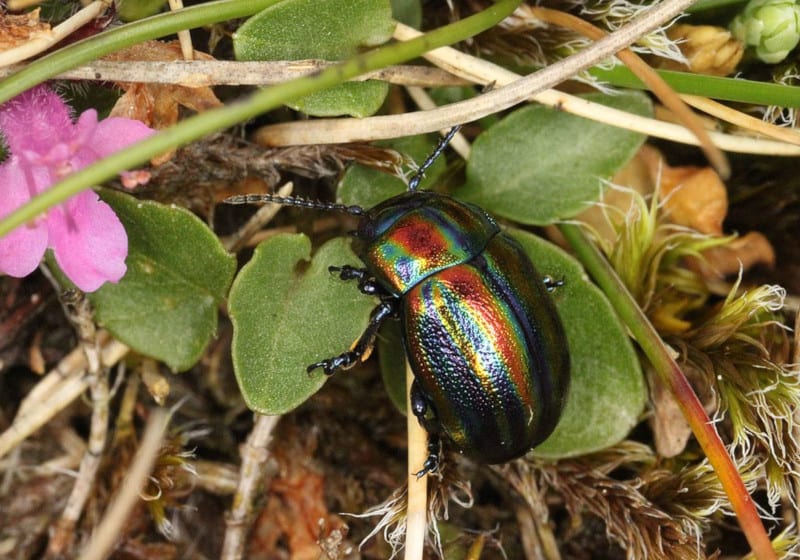In the wide horizontal photo, an insect resembling a June bug or beetle takes center stage on a green leaf amidst a richly detailed natural ground setting. The beetle's body showcases a mesmerizing metallic and iridescent sheen, featuring colors such as red, green, blue, yellow, orange, and faded streaks of yellow and dark red, along with distinctive black legs and antennae. The background reveals a complex tapestry of thin vines, twigs, and grass roots, interspersed with variously colored leaves and stems. In the upper left corner of the image, a small pink flower petal adds a splash of color. Shadows and dark patches are scattered across the ground, contributing to the image’s depth and texture. The photograph captures the beetle from a slightly elevated angle, offering a detailed view of its shiny, segmented body and intricate positioning of its legs as it perches on the leaf, emphasizing the insect’s small size relative to its surroundings.